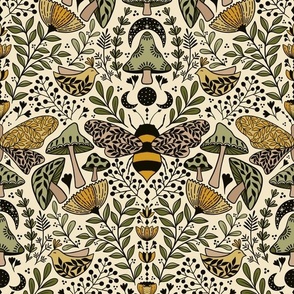The image is a square piece of art, resembling a modern rendition of a vintage wallpaper pattern with a muted color palette primarily consisting of pale olive green, yellow, light tan, black, and mauve on a light yellow background. At the center, a large black and yellow striped bee is prominently featured with light brown wings that have a black leaf print on them. Above the bee, the moon is depicted in various phases, alongside a green mushroom with a brown stem and another moon cycle. Surrounding these central elements, the print includes an array of intricately designed birds and leaves. The birds are yellow with detailed black leaf patterns on their wings and breasts, reminiscent of fern fronds. Scattered throughout the pattern are a variety of bright yellow upward-pointing flowers and sprigs of black berry-like branches, possibly elderberries. The leaves vary in shape, some are typical ovals while others are more pointed, with the majority being green. Additionally, each side of the image shows a yellow butterfly wing with a leaf pattern, transitioning to brown with the same black leaf design beneath. The entire composition combines these elements into a cohesive and repetitive botanical design, striking a balance between detailed intricacy and modern simplicity.